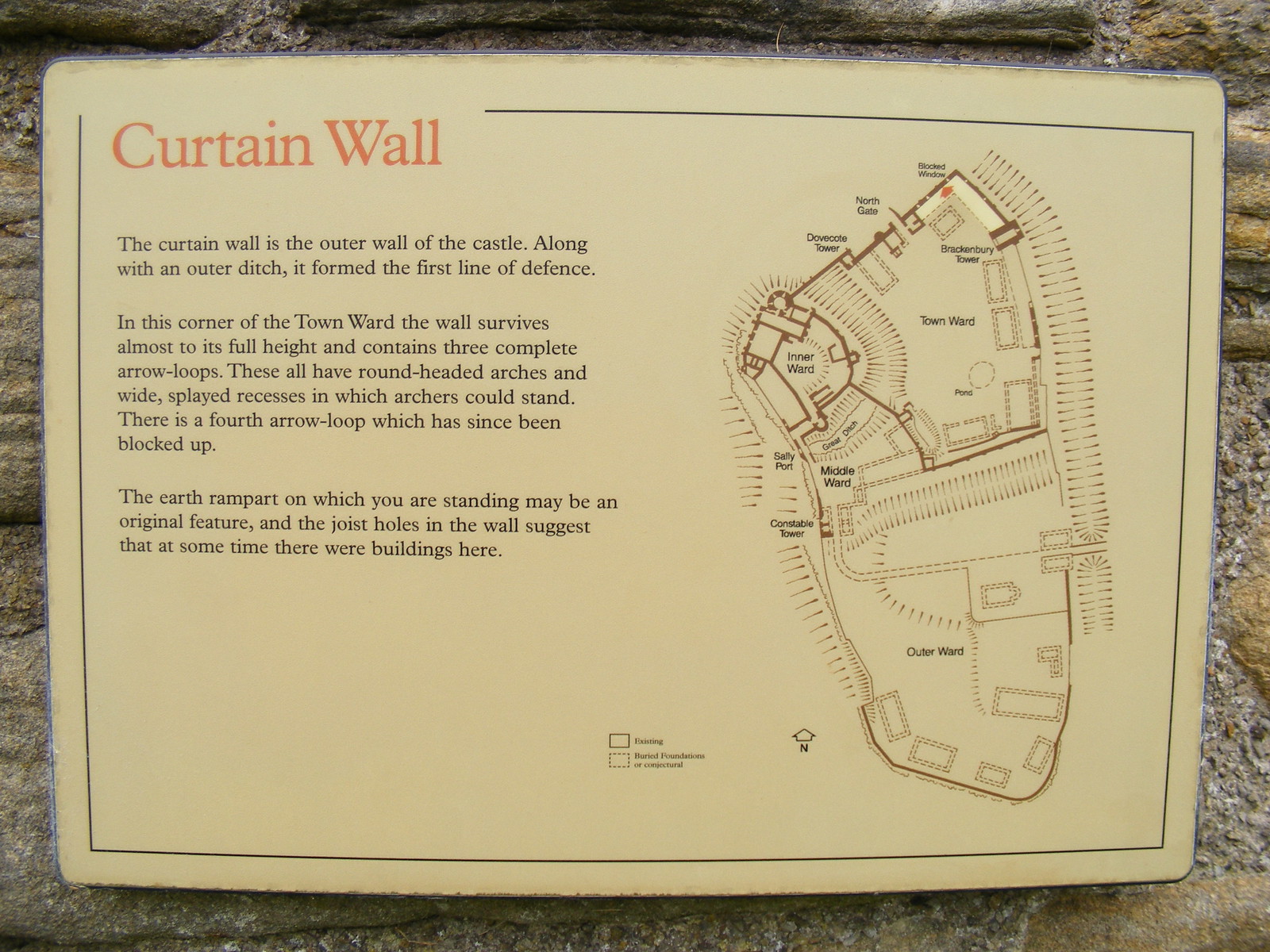The image depicts a laminated informational placard mounted on a stone wall with gray, grainy mortar. The rectangular placard has a thin black border and a beige background. In the upper left corner, bold orange text reads "Curtain Wall." Below this heading, smaller black text explains that the curtain wall is the outer wall of the castle and, along with an outer ditch, formed the first line of defense in the corner of the Town Ward. The text details that this section of the wall survives almost to its full height and contains three complete arrow loops with round-headed arches and wide splayed recesses where archers could stand. Additionally, it mentions a fourth arrow loop that has been blocked up. It also notes that the earth rampart on which viewers stand may be an original feature, and that joist holes in the wall suggest buildings once stood nearby. On the right side of the placard, there is an overhead map of the area, highlighting sections labeled Town Ward, Outer Ward, Middle Ward, Sally Port, Constable Tower, Dovercoat Tower, North Gate, Blocked Window, and Brackenberry Tower.